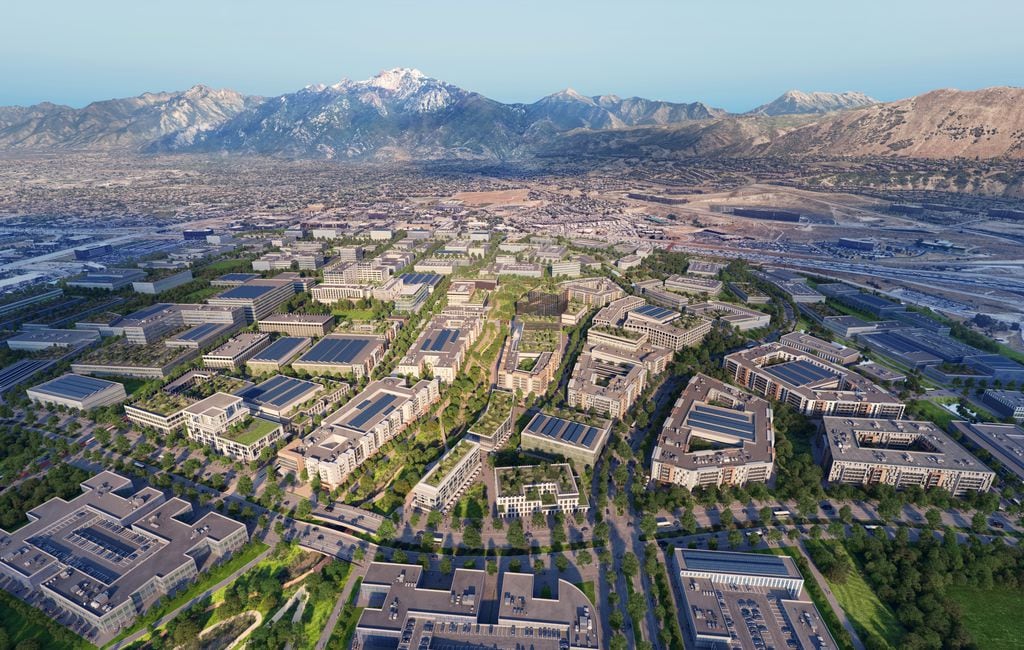A breathtaking aerial view captures the expansive layout of a bustling city nestled at the foot of a snow-capped mountain range. The image showcases numerous sizable buildings, primarily office and apartment complexes with flat roofs, many adorned with solar panels. The roofs are otherwise largely unadorned, except for some air conditioning equipment. Streets lined with non-indigenous trees weave through the cityscape, including a prominent road cutting through the foreground from left to right. The lower right-hand corner reveals verdant green spaces, hinting at parks or communal areas amid the urban sprawl. In the distance, the city's dense cluster of buildings stretches towards towering mountains, which flaunt their snowy peaks on the left side. The scene is enveloped by a brilliant, cloudless blue sky, suggesting a crisp day, possibly in early spring.